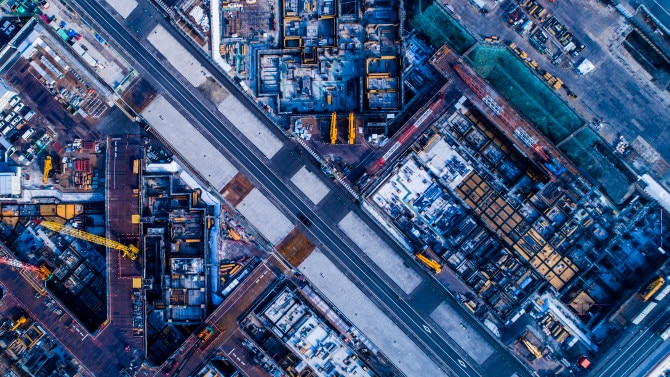The image is an aerial shot of what appears to be a sprawling industrial area, possibly a shipping yard or large factory complex. Dominated by hues of blue, gray, green, and yellow, the photograph captures a detailed view of the expansive setting from a high altitude. Running diagonally through the image are two main roadways, distinctly marked in blue and white, intersecting amidst a network of smaller roads. Surrounding these roadways are numerous buildings and structures, likely part of the industrial operations, along with what seems to be parks or open spaces. The upper right section of the image reveals several cranes and vehicles, indicative of heavy machinery at work, while additional cranes are scattered across other parts, contributing to a sense of ongoing construction or activity. The layout and the mechanical elements give an impression reminiscent of a giant circuit board, marked by an array of cranes, potential bridges under construction, and various pieces of large machinery without visible roofs.